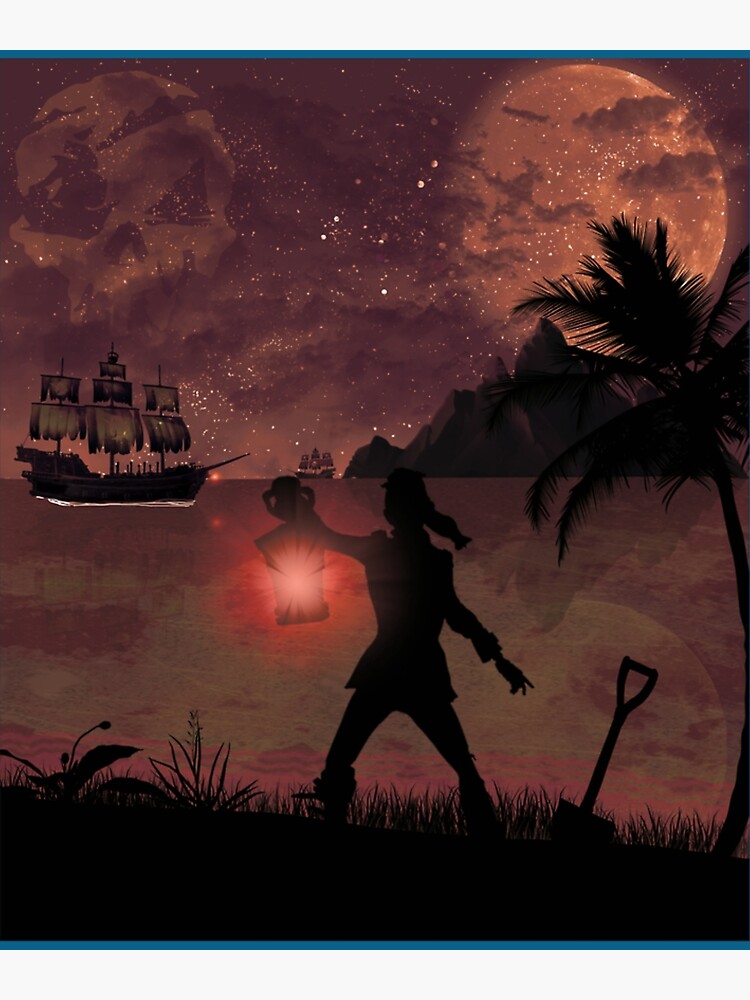In this richly detailed fantasy painting, set in a vertical rectangular frame, we see a multi-color artistic piece themed around pirates. The scene is devoid of a definitive background and features a faint blue border on the top and bottom edges. The upper left corner of the artwork showcases a spectral human skull with a ship forming one of its eyes and an angry triangle eye on the other, its lower jaw ominously missing. Scattered stars pepper the sky, and the top right houses a partially obscured moon with wispy clouds drifting by.

Central to the image, we observe a distant ship sailing the waters, its tattered sails catching the breeze. Closer to the viewer, on the center left, stands another pirate ship with flags fluttering. Dominating the foreground is the silhouette of a pirate standing on the shore, one hand holding a lit red lantern outward with a glow illuminating his surroundings, and the other next to a shovel planted firmly in the ground, hinting at recent or impending treasure burying. A variety of colors, including light purple, dark purple, black, off-white, orange, and lavender, enrich the scene.

A palm tree and distant mountain peaks or rock walls frame the right side of the composition, grounding this night-time coastal tableau in natural elements. The pirate is surrounded by grass and plants, adding texture to the shore where he stands. This meticulously crafted image captures the adventurous and mysterious essence of pirate lore with a wealth of vivid and dynamic details.